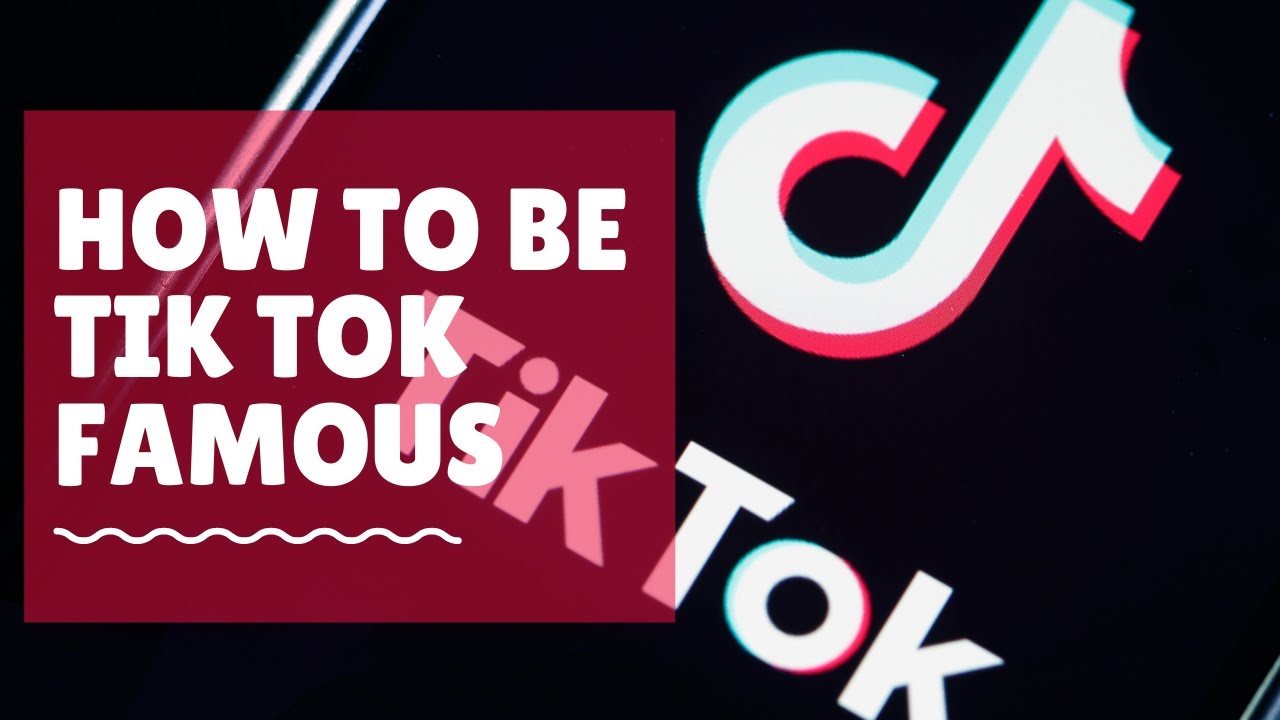The image features a stark black background prominently displaying the TikTok logo. The logo consists of a stylized white musical note resembling a capital 'T' merged with an 'O' that creates a sweeping, dynamic upward and rightward arc. Beneath this emblem, the word "TikTok" is inscribed in bold white text. To the left of the logo, there is a semi-transparent, maroon-colored square with the phrase "How to be TikTok Famous" boldly written in white capital letters. Underneath the maroon square, a continuous squiggly line meanders across the image, creating a rhythmic pattern of up and down curves. The line adds a playful element to the design, enhancing the visual appeal against the dark background.